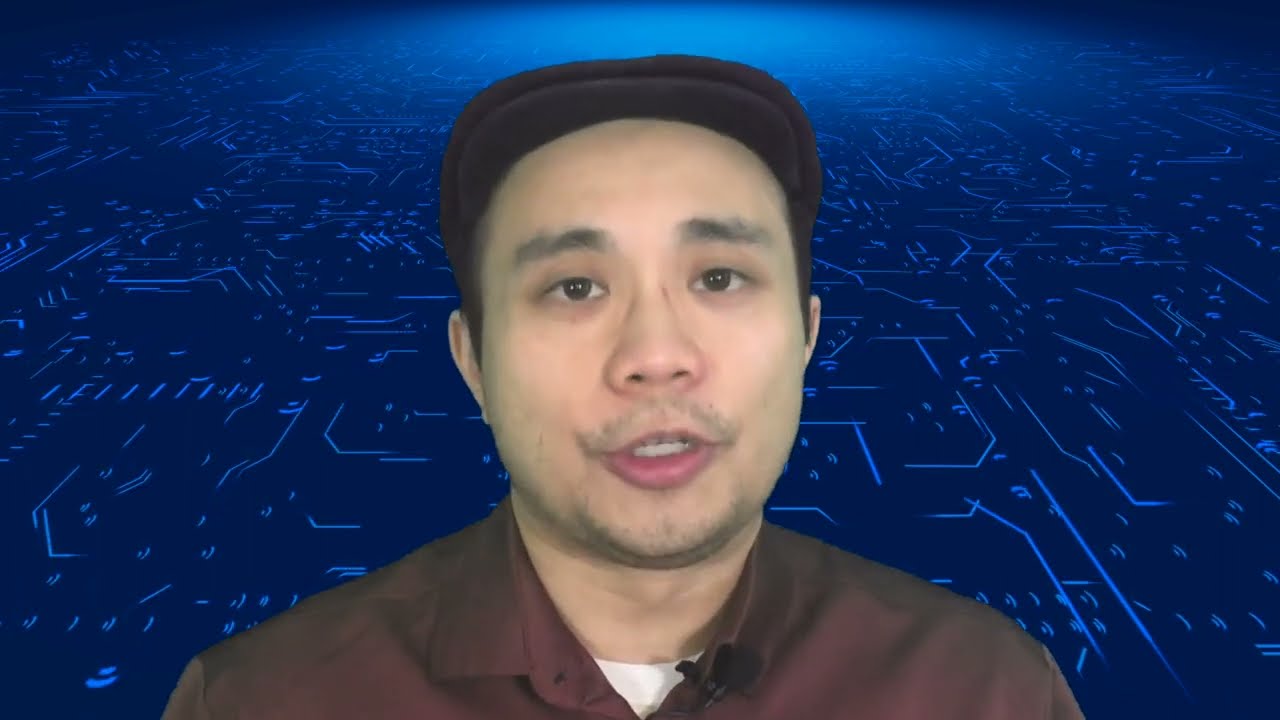This image features an Asian-looking man during a live stream or video call, possibly on social media or a video meeting platform. He has a brown hat and a brown buttoned shirt that is open at the collar, revealing a white undershirt. His face shows some beard stubble and a slight mustache, with bushy, somewhat triangular eyebrows. His mouth is open, and you can see some of his teeth, indicating he is speaking. The background is a striking blue and dark blue with highlights, resembling the intricate design of a computer chip or motherboard, giving off a cyberpunk or futuristic aesthetic. The blue background appears animated and illuminated by a light source at the top, creating a vivid and dynamic backdrop for the man who seems to be engaging his audience.